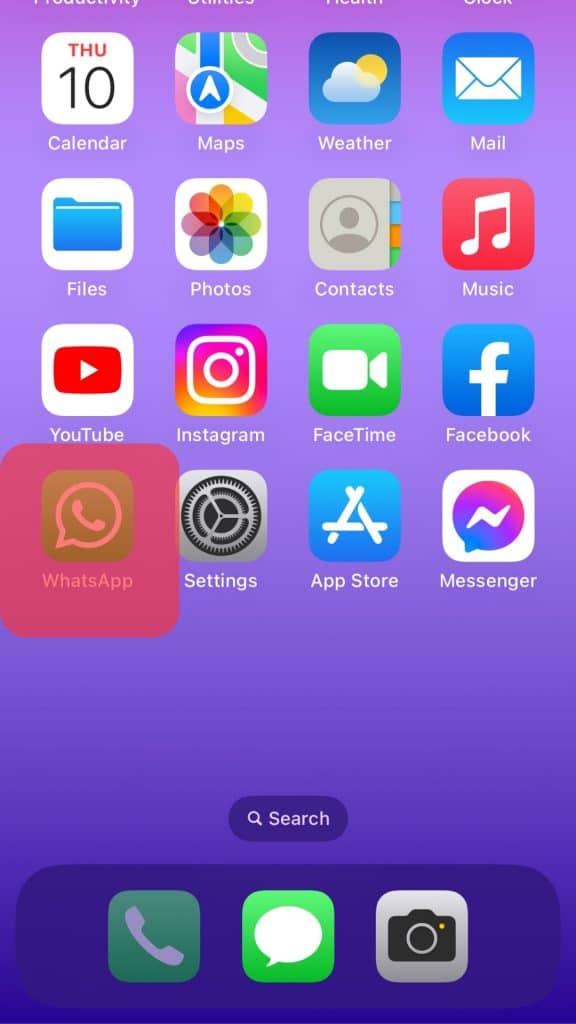Here is a refined and detailed caption for the image based on the provided description:

"This image is a cropped screenshot of an Apple iPhone's home screen, excluding the very top portion. The screen displays 16 app icons arranged in a 4x4 grid. Notably, the bottom row consists of icons such as WhatsApp, which is highlighted by a red semi-transparent overlay box, possibly to draw attention to it. Below this grid, three icons are located in the dock: the phone icon on the left, the chat/text message icon in the center, and another phone icon on the right, which appears grayed out, suggesting it is currently unusable. The background of the screen is a gradient of purple, transitioning from a light shade at the top to a darker hue at the bottom."